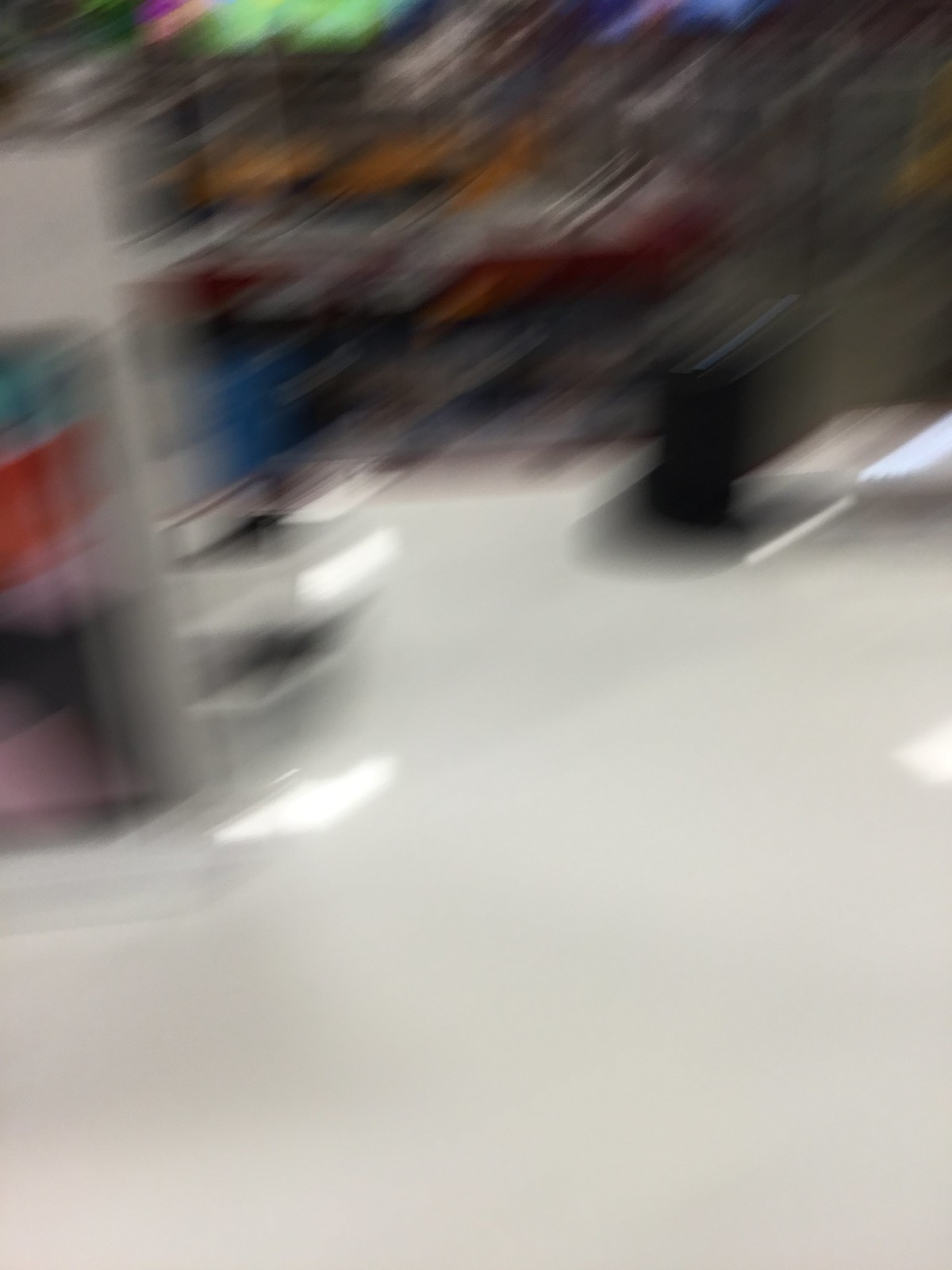In this extremely blurry image, you can barely distinguish various shapes and colors. The bottom half of the image appears predominantly white, possibly indicating a floorboard or the floor of a retail store. In the upper left corner, there's a vague outline of what seems to be a white shelf. Extending from the front side of this shelf are indistinct line shapes that might represent additional shelves, with light reflecting off their surfaces. The background is a kaleidoscope of colors, including yellows, reds, blues, and many dark tones, creating an overall cluttered appearance. Scattered lights on the ground suggest reflections off a glossy floor, contributing to an environment that’s hard to clearly identify.